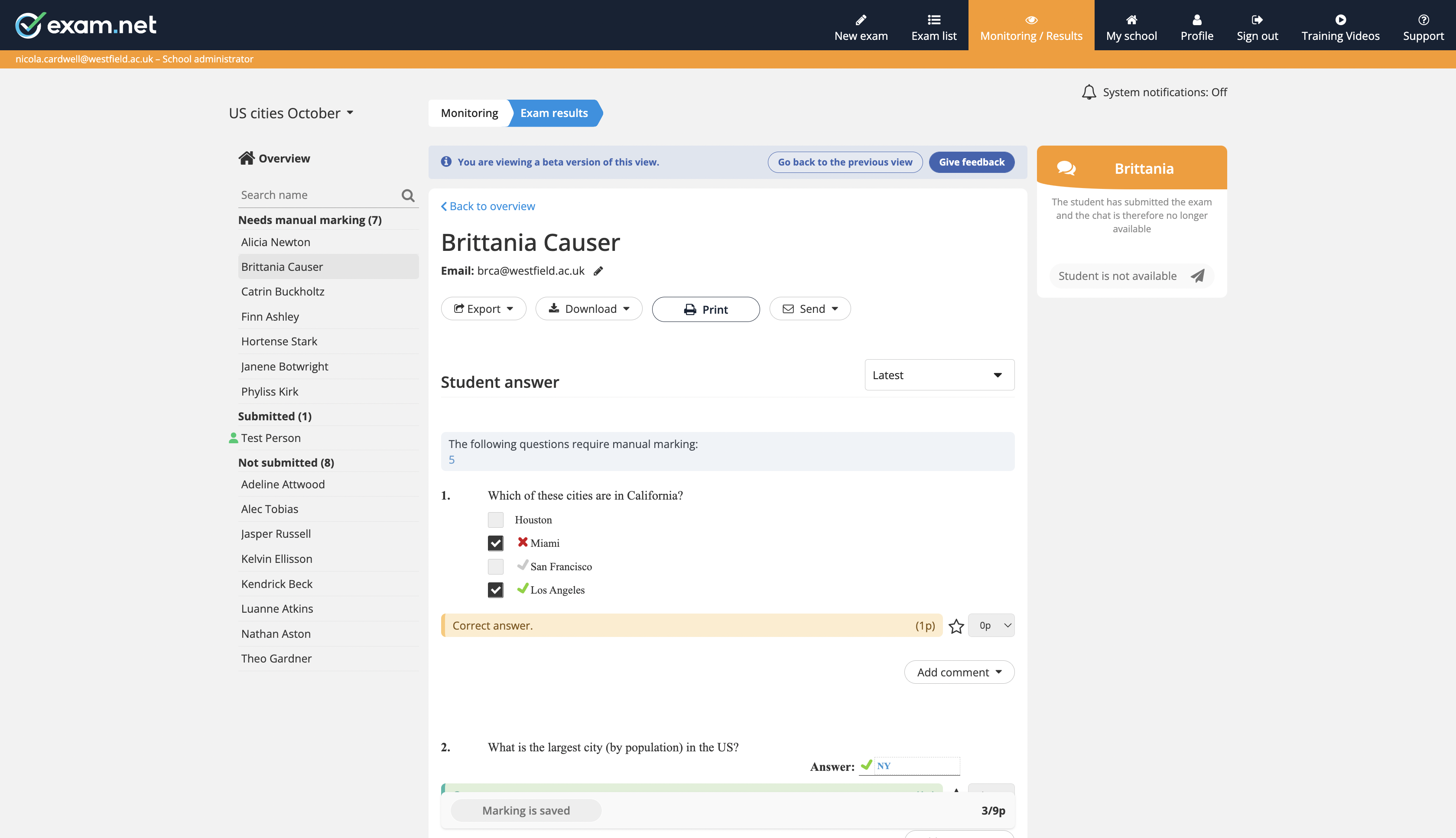**Detailed Caption:**

This image is a detailed screenshot from the website Exam.net. The interface shows various headings at the top of the page, including 'New Exam,' 'Exam List,' 'Monitoring & Results,' 'My School,' 'Profile,' 'Sign Out,' 'Training,' and 'Business Support.' The 'Monitoring & Results' tab is currently selected.

The main section of the page displays "Monitoring and Exam Results" with a notification that the viewer is using a beta version of this view, along with the options to "Go back to previous view" or "Give feedback."

The page appears to be specifically for a user named Britannia Calzer. Her email address is displayed, along with buttons for exporting, downloading, printing, and sending the information. Below this, the page lists student answers and highlights questions that require manual marking.

One question displayed is: "Which of the following cities is in California?" The options provided are Houston, Miami, San Francisco, and Los Angeles. The student answered Miami and Los Angeles. Miami is marked incorrect, while Los Angeles is correct. San Francisco was another correct option that the student missed.

Another question reads: "What is the largest city by population in the U.S.?" The correct answer provided was New York, and the student answered this correctly.

The left side of the page shows a list of other students, indicating this is a comprehensive monitoring tool for managing exam results.